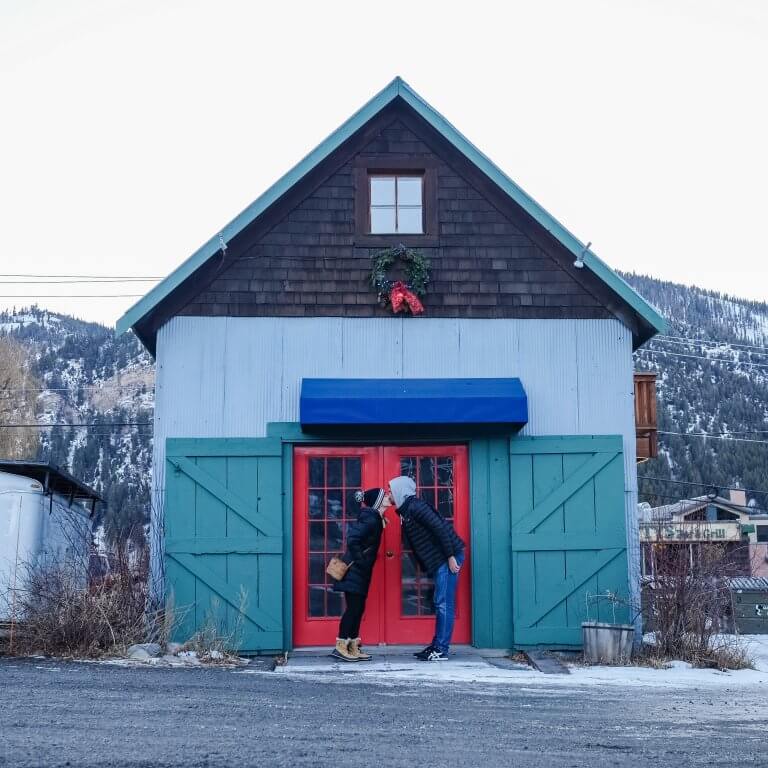**Caption:**

A charming house, adorned with three distinct colors, stands as a picturesque backdrop for a romantic moment between a couple. The upper section of the house features a window with white blinds, framed by brown shingles, and complemented by a festive Christmas wreath hanging underneath. Directly below, the exterior is painted white, resembling smooth wood panels. The entrance area is a vibrant assembly of colors, including a blue awning that shelters a pair of green barn-like doors and a striking red door in the center.

In front of this colorful facade, a couple shares a tender kiss. On the left, the woman, dressed entirely in black with brown shoes, stands slightly shorter than the man on the right. He contrasts her attire with a hoodie beneath a black jacket paired with blue jeans. The setting is enhanced by the majestic mountains in the background and the lush shrubbery adorning the front of the house, creating a serene and heartwarming scene.